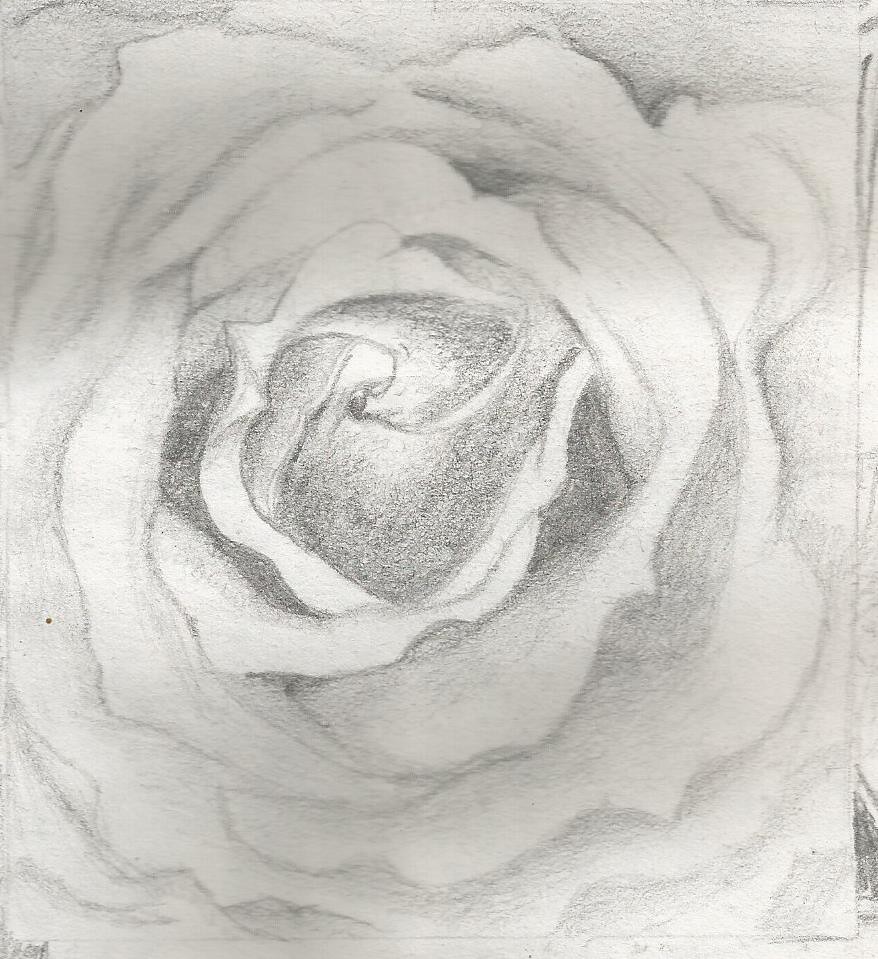This detailed pencil sketch depicts a rose in full bloom, rendered entirely in shades of gray without any color. The artwork is signed in the bottom left-hand corner with a small signature that appears to read "Jessa," although the exact name is not entirely clear. The artist has paid meticulous attention to the intricate details of the rose, particularly the curled petals and the shaded, tightly wound center bud. The sketch fills the entire sheet of paper, leaving no background or surrounding elements. The petals are incredibly detailed, with delicate, natural curls and subtle shading between the layers, giving the rose a lifelike depth and texture.